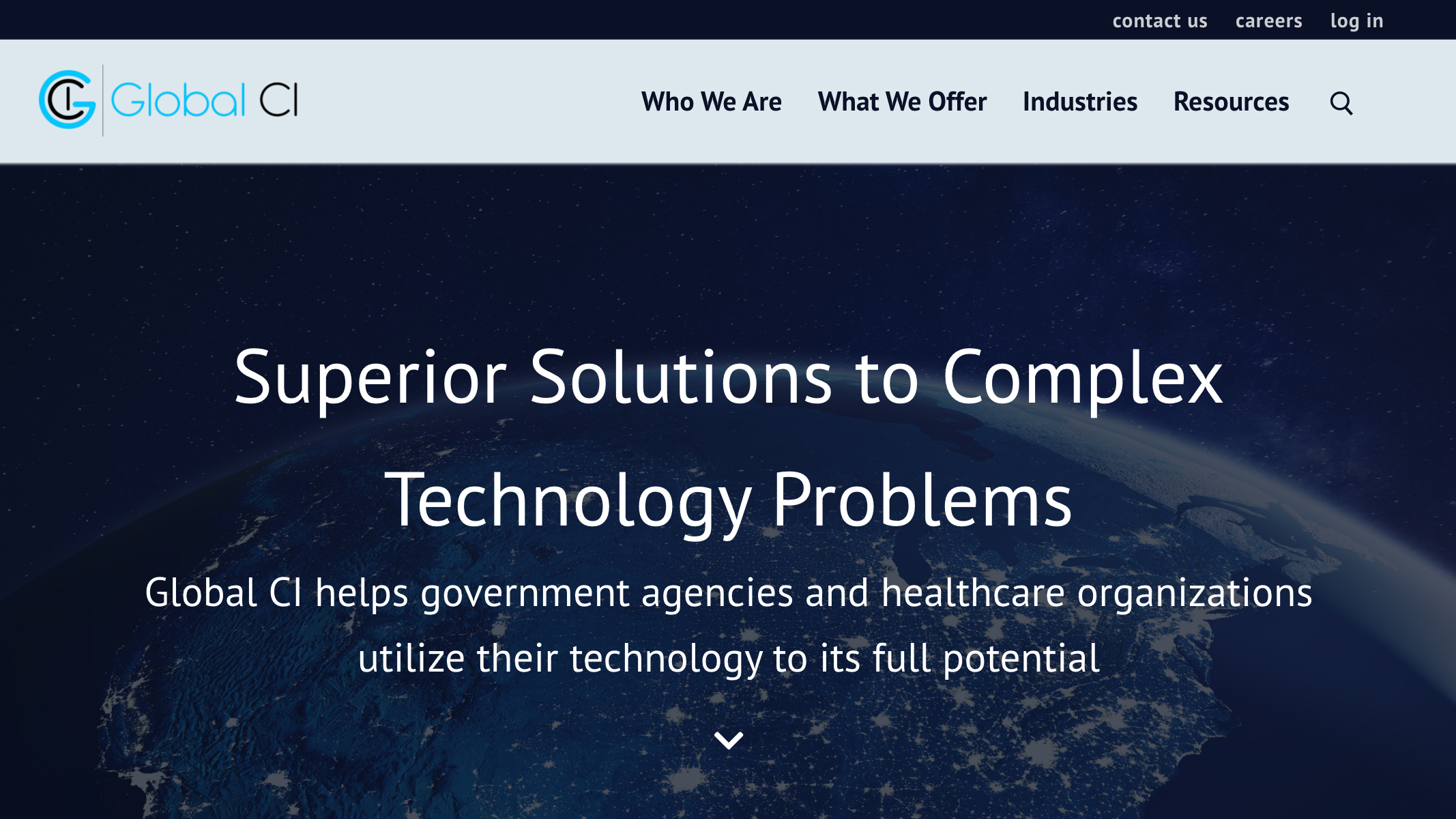The image appears to be a screenshot of a website interface with various UI elements. In the upper left corner, set against a light blue background, the text "Global CI" is prominently displayed. Adjacent to this, to the right, is a navigation menu featuring the items: "Who We Are," "What We Offer," "Industries," "Resources," and an icon resembling a magnifying glass, suggestive of a search function, is positioned in the upper right corner.

Below this, a darker blue section extends across the screen. A partially visible background image seems to depict planet Earth from space, adding a thematic touch to the website. Superimposed on this background, larger white text reads, "Superior solutions to complex technology problems." Below this headline, smaller white text states, "Global CI helps government agencies and healthcare organizations utilize their technology to its full potential." A downward-pointing arrow icon, also in white, is present underneath the text.

Additionally, situated above the light blue area, a slimmer black bar spans the top of the page. Within this bar, on the right side, white text provides links labeled "Contact Us," "Careers," and "Login."